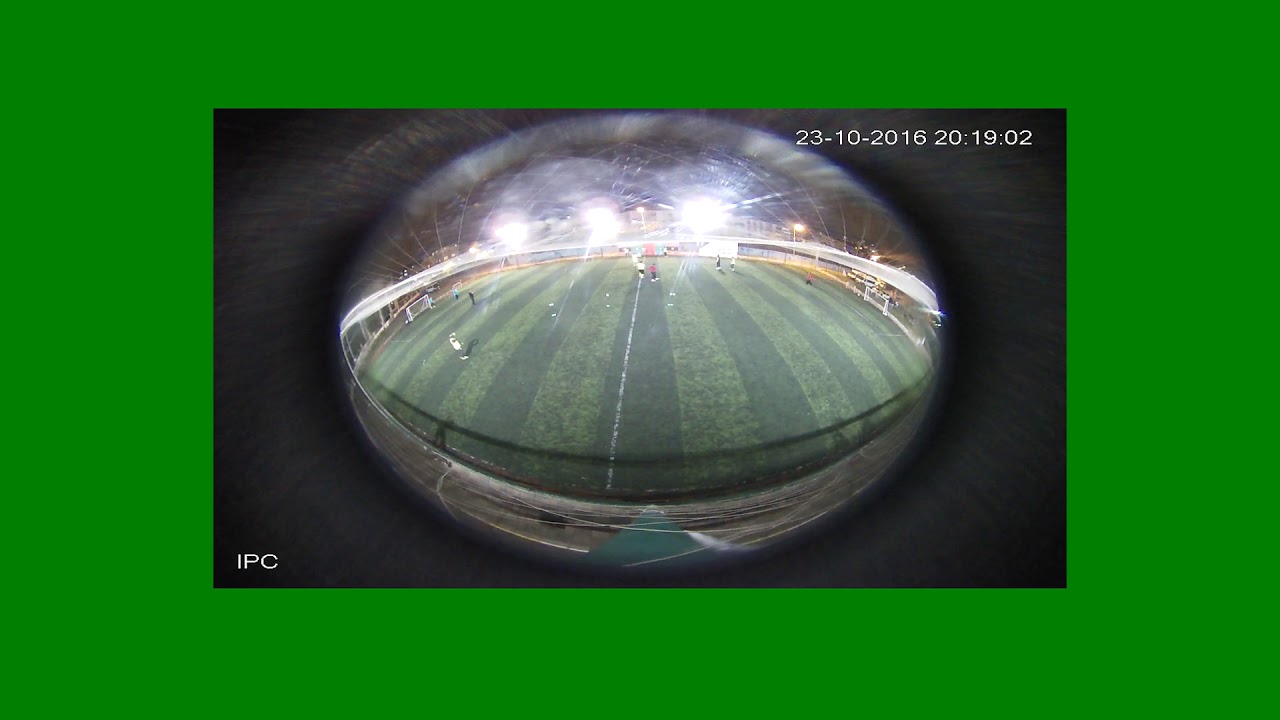The photograph captures a sports field through a fisheye lens, presenting a unique, distorted perspective. The central circular image touches both the top and bottom edges of the frame. It shows a green soccer field with alternating patches of light and dark green grass, a white line running down the center, and white goals on either side. The field is illuminated by three stadium lights near its center, which obscure some details. The distant figures on the field appear indistinct, adding to the mysterious ambiance. Surrounding this circular image is a dark, metallic black background with faint radiating lines. The entire image is bordered by a thick green frame, thicker on the vertical sides. In the bottom left corner, the letters "IPC" are visible in white text, while the top right corner displays the date and time "23-10-2016 20:19:02" in white font. The composition resembles a glass marble or spherical object containing an aerial view of the soccer field.